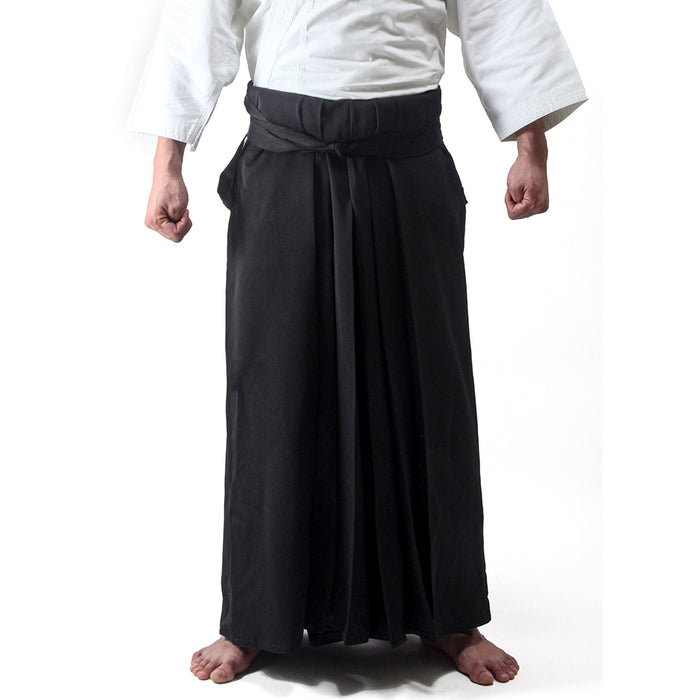The image depicts the lower half of a person, likely male, standing in a prepared stance. The individual is wearing a white martial arts jacket with long, baggy sleeves, possibly akin to a chef's coat, indicating a disciplined or professional background. His hands, which are bare and clenched into fists with thumbs inside the fingers, are held away from his sides, suggesting readiness for combat or demonstration. Below, he dons a long, black skirt with potential transparency at the very bottom, hinting at a layered design or solid area underneath. A black belt cinches the waist of the skirt, further implying martial arts attire. The person's feet are barefoot, solidifying the martial arts context, and the stance is notably wide, reinforcing a posture of alertness and readiness to engage.